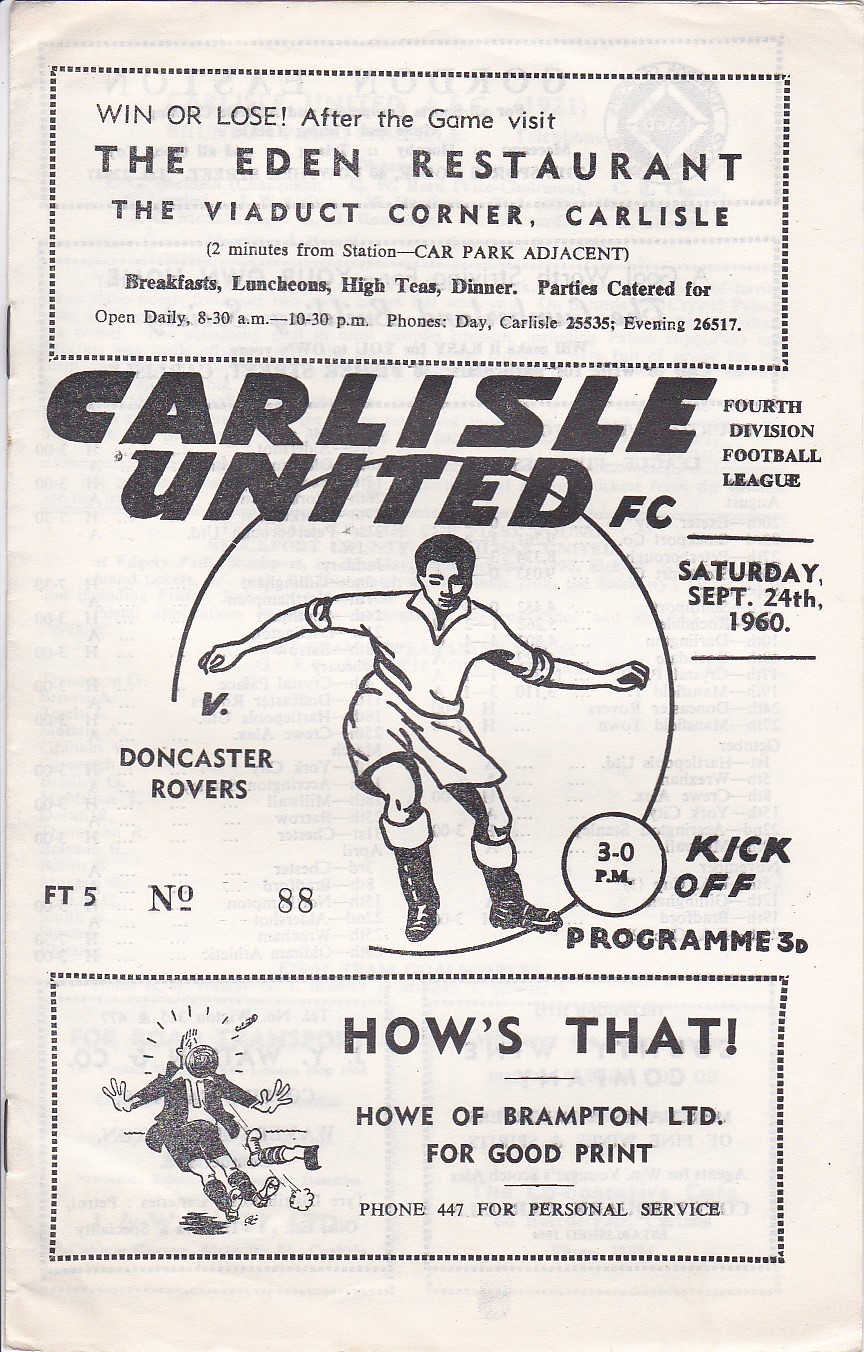The image depicts an aged and close-up photograph of a vintage English football match program cover from Saturday, September 24th, 1960, featuring Carlisle United FC versus Doncaster Rovers. The program is predominantly black and white, printed on off-white, creamy, textured paper. At the center, bold black text announces "Carlisle United FC" with "versus Doncaster Rovers" just below it. Additionally, there is a prominent illustration of a footballer, clad in black boots and a white kit, located centrally within a circular design. The top advertises the Eden Restaurant, encouraging match-goers to visit "Win or lose, after the game," providing details like the location at the Viaduct Corner in Carlisle, the proximity to the station, and operational hours from 8:30 a.m. to 10:30 p.m., along with contact phone numbers. The bottom advert features How's That How of Brampton Limited, a printing company, emphasizing their quality print services and listing a contact number for personal service.